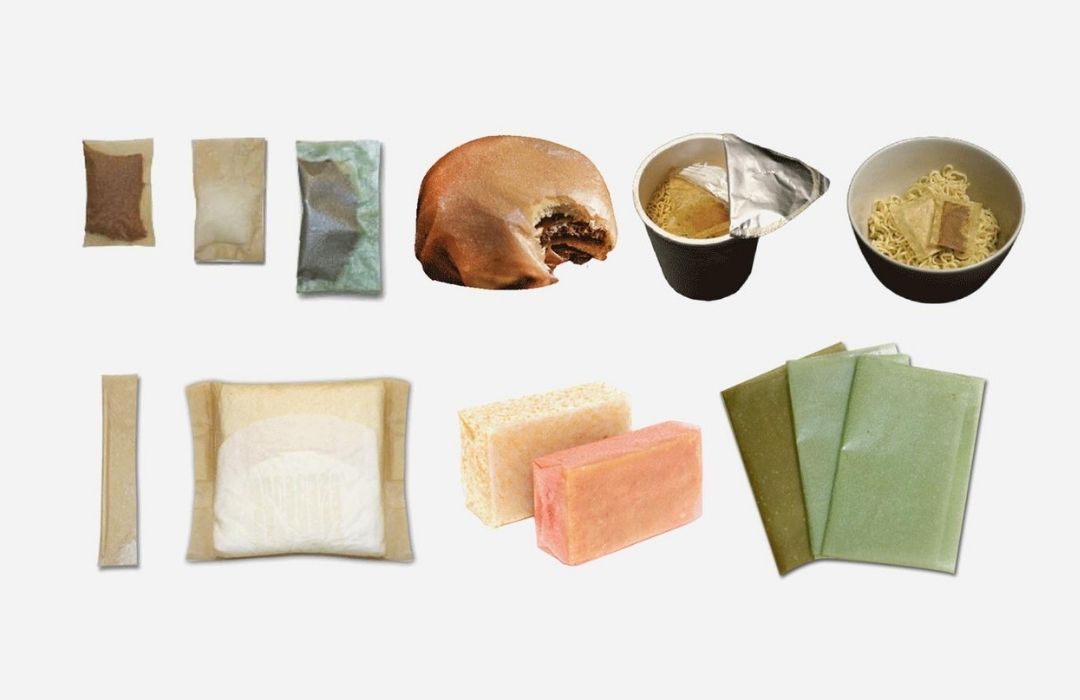The image displays a curated arrangement of ten food items, meticulously laid out on a white background in two horizontal rows, with individual items presented within varied packaging. Starting from the top-left: a small rectangular light brown packet, possibly holding a brown and fine substance like tea or powder; a slightly larger packet containing a white, powdery substance that might resemble salt or sugar; a shiny, bluish-green packet containing a brown paste or similar substance; and a spherical bun with a chocolate-like exterior, a bite taken out, revealing a dark filling inside. Further right is a navy blue cylindrical container with a white rim, its foil top peeled back to reveal a brown powder inside, possibly a soup or drink mix. Adjacent is a larger blue bowl filled with white ramen noodles and two of the aforementioned packets. Moving to the bottom-left: an elongated vertical rectangular packet; a larger brownish packet with a white substance, possibly tofu. Next, two brick-like items: one white and one light pink bar that may resemble soap or fish slices. The final grouping features three green packets, fanned out in different shades of green, possibly representing various rice or paper wrappers. These individual components seem to collectively form a deconstructed meal package, providing an intriguing visual and detailed insight into the arrangement of various food items.